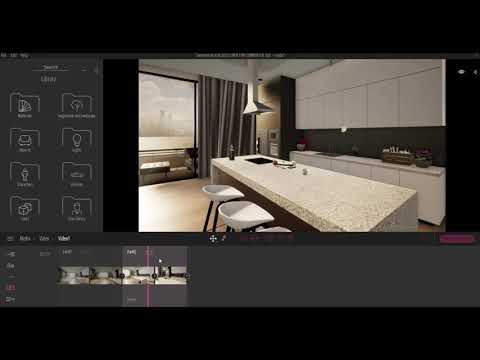This image appears to be a detailed screenshot of a computer-generated kitchen design, likely created using an interior design application or video editing software. The screen has black borders on the top and bottom, and the left-hand side features a gray vertical banner displaying white outlines of file folders. The main picture frame showcases a modern, upscale kitchen scene, illuminated by a large window that seems to overlook either an ocean, lake, or field, enhanced by dark gray drapes fully drawn to one side.

Central to the design is a long granite island with a sink cutout and three white bar stools arranged in front. Above the island, an exhaust hood hangs elegantly. The kitchen backdrop includes a dark wall, possibly dark blue or black, adorned with white cabinetry both above and below. The upper section features a header and the lower section accents with a countertop adorned with baskets and other decorative items. The cabinetry and overall design maintain a sophisticated aesthetic with a mix of earth tones, wood, marble, black, white, gray, and occasional red hues, contributing to the luxurious and modern feel of the space.